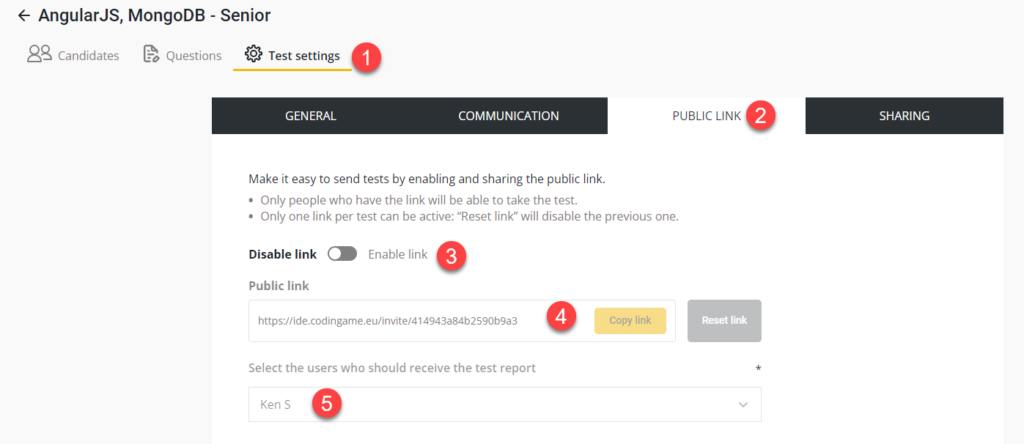A screen capture of a monitor displays a detailed interface with multiple elements and labels. 

The background is slightly off-white, and in the top-left corner, "AngularJS" is prominently displayed in bold font. Adjacent to it, "MongoDB-theme" is written with a black arrow pointing to the left. Below this, on the left, there is a light gray icon depicting two people, labeled "candidates." Next to it, there's a page labeled "questions." The "settings" section, highlighted by a yellow line, is noted in black text. Adjacent to this section is a red circle with the number "1" inside.

Beneath this area is a horizontal black banner divided into four tabs: "General" and "Communication" are in white on black but not active, while "Public Link" is highlighted in white and contains a red circle with a white "2" inside. The last tab, "Share," appears in white text on a black background. 

The content area below the banner contains a white text block explaining, "Make it easy to send tests by enabling and sharing a public link. Only people who have the link will be able to take the test. Only one link per test can be active. Reset link will disable the previous one." Below this text, bold text states "Disable link" (which is turned off) and "Enable link" (to the right of which is a red circle with the number "3").

Below this, the public link "identity.edu" is displayed in a URL window, accompanied by a red circle with the number "4." To the right of the URL field, there is a yellow button labeled "Copy link" and a gray button labeled "Reset link."
 
Further down, in gray text, instructions read, "Select the user who should receive the test report." Accompanying this is a field with a drop-down arrow on the right. The name "Ken S." appears in light gray on the left of the field, and a red circle with the white number "5" is positioned to its right.